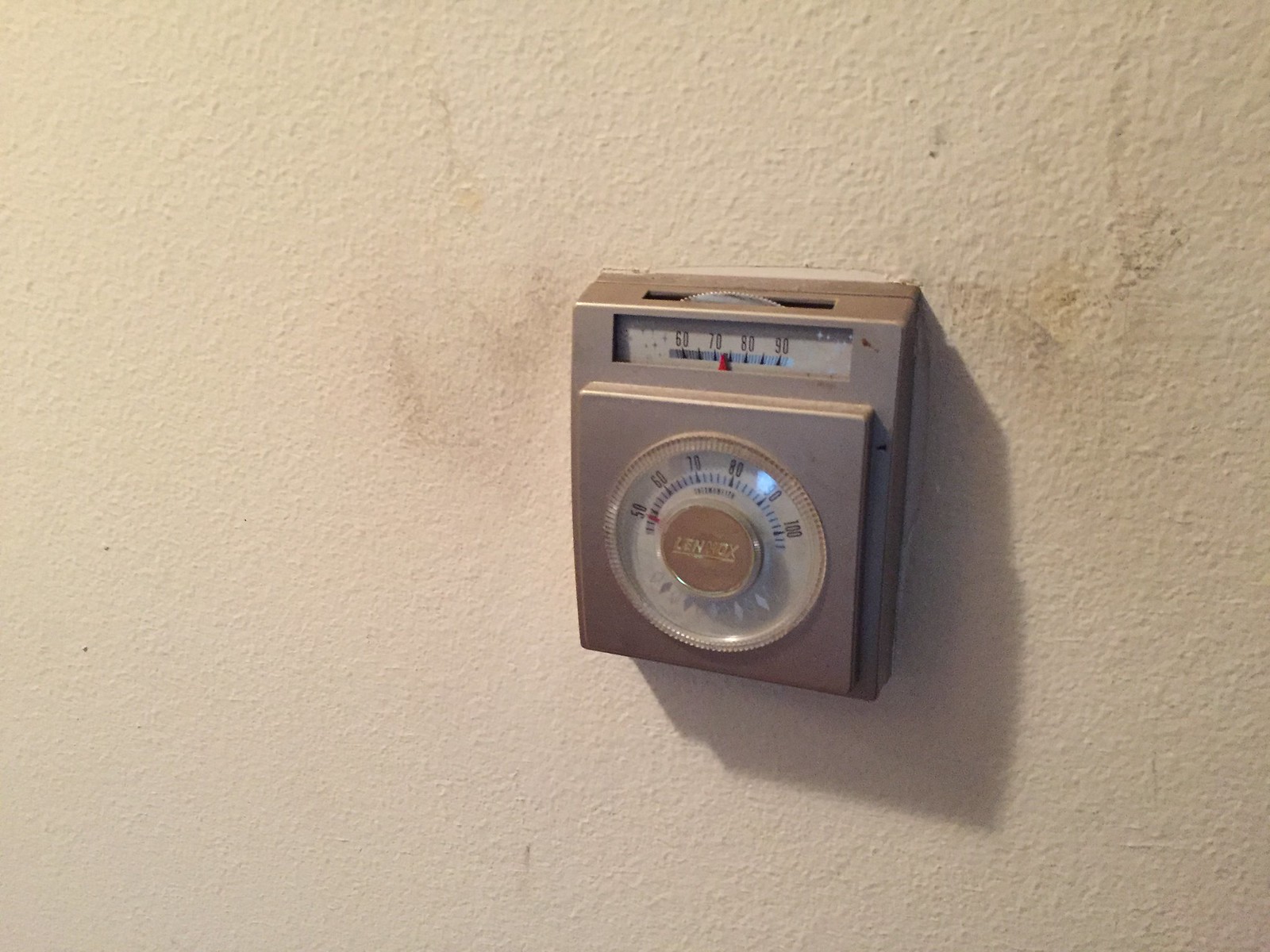A brightly lit room reveals a prominently textured white wall that bears numerous stains and marks, ranging from brown and yellow stains to black smudges. Casting shadows upon the wall is an old, silver thermostat with a distinctly retro design. This dated device features a prominent round dial on its front. Centrally positioned on the thermostat is an embossed logo that reads "LENNOX" in uppercase letters. The rotary dial at the bottom spans a range from 50 to 100 degrees Fahrenheit, while a cut-out circular dial on the top, moving left to right, goes from 60 to 90 degrees. The thermostat currently displays a reading of 74 degrees, indicated by a conspicuous red arrow.